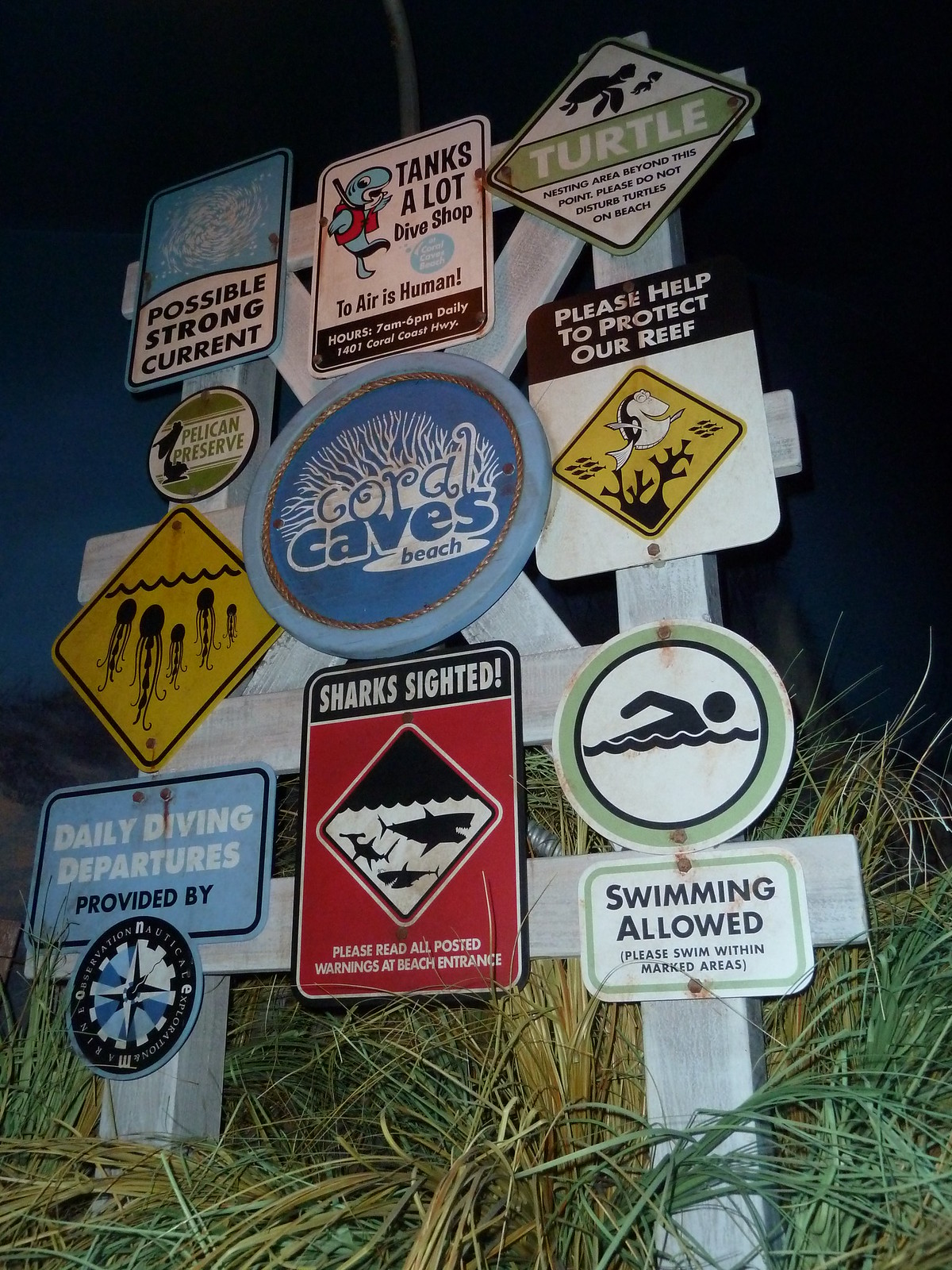The image showcases a wooden signpost anchored in a grassy area with green and brown grass surrounding its base. The signpost is constructed from white wooden planks arranged horizontally and vertically, with two diagonal planks crossing in the middle for added support. Affixed to this wood frame is an eclectic collection of various metal signs, creating a visually engaging collage.

Prominently centered is a circular blue sign with white line art depicting coral, labeled "Coral Caves Beach." Surrounding this centerpiece are numerous informative signs. At the top, another sign warns of a "Possible Strong Current" with an illustration of swirling water. Nearby, a playful advertisement for a dive shop reads, "Tanks a lot, dive shop. To air is human," and provides hours of operation and its location at 1401 Coral Coast Highway. To the right of these is a sign noting "Turtle Nesting Area Beyond This Point. Please Do Not Disturb Turtles on the Beach," accompanied by a turtle illustration.

Additional signs include a warning about "Pelican Reserve," an advisory to "Please Help Protect Our Reef," and notice regarding jellyfish presence in the water. Mid-frame, a yellow sign with an octopus silhouette heads towards the surface under the caption "Daily Diving Departures Provided By" and features an unreadable compass emblem. Notably, a red and black sign alerts beachgoers to "Shark Sighted" in the area, advising to "Please Read All Posted Warnings at Beach Entrance." Lastly, a circular sign indicates "Swimming Allowed. Please Swim Within Marked Areas," with an illustration of a person swimming.

The overall composition is set against a backdrop that is noticeably dark at the top, possibly hinting at an evening sky or shade from surrounding foliage. The dense arrangement of signs provides crucial information about the local marine environment and safety guidelines for visitors.